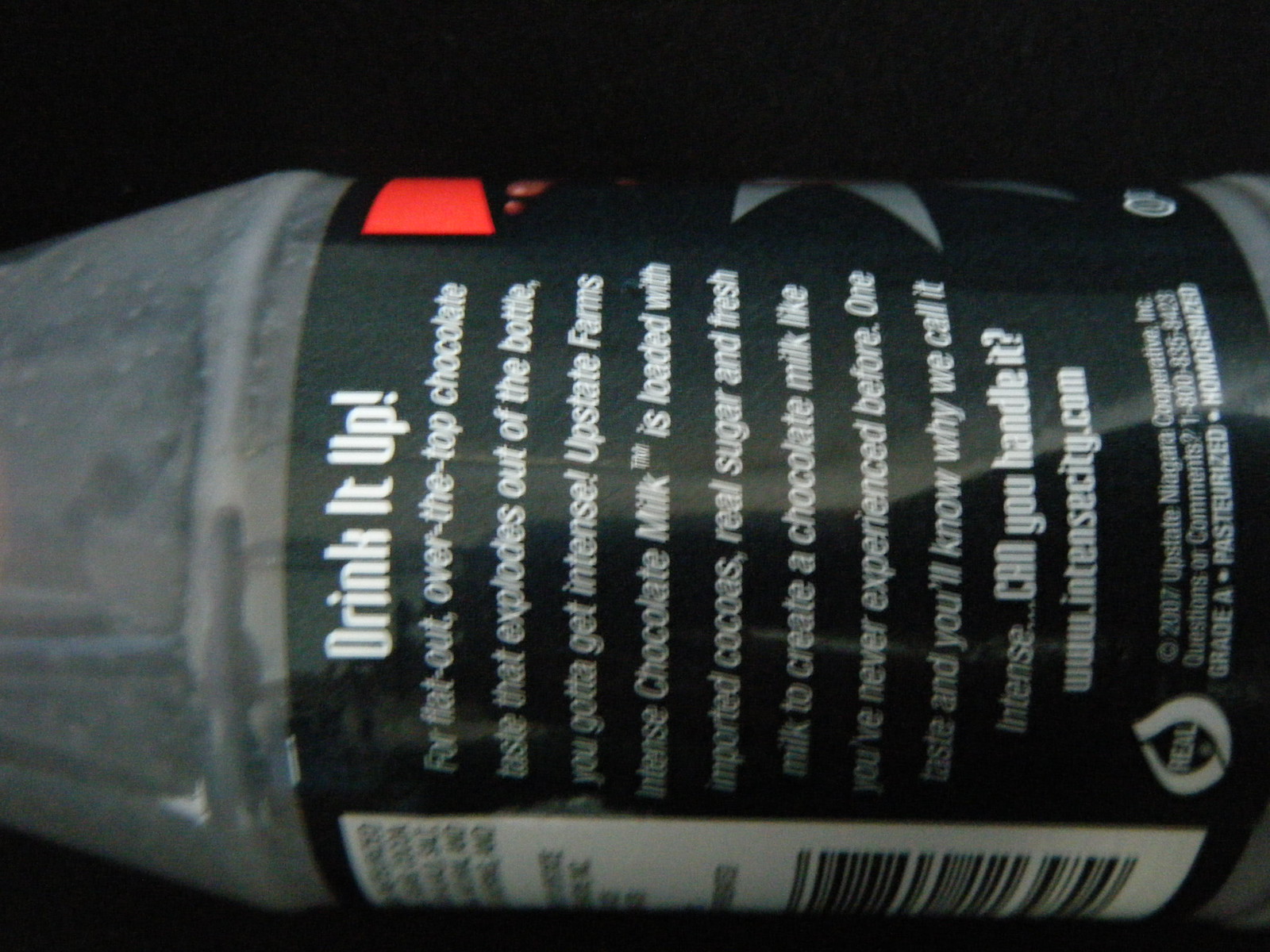The image features a horizontally positioned bottle that stretches from the left to the right edge of the frame. A small strip of black background is visible at both the top and bottom. The bottle's label, displaying the back side, prominently features the brand's marketing slogans. The text reads: "Drink it up. For flat out, over the top chocolate taste that explodes out of the bottle, you gotta get intense. Upstate Farms Intense Chocolate Milk™ is loaded with imported cocoa, real sugar, and fresh milk to create a chocolate milk like you've never experienced before. One taste and you'll know why we call it intense." The focus is on the rich details of the label, aiming to convey the exceptional taste and quality of the beverage.